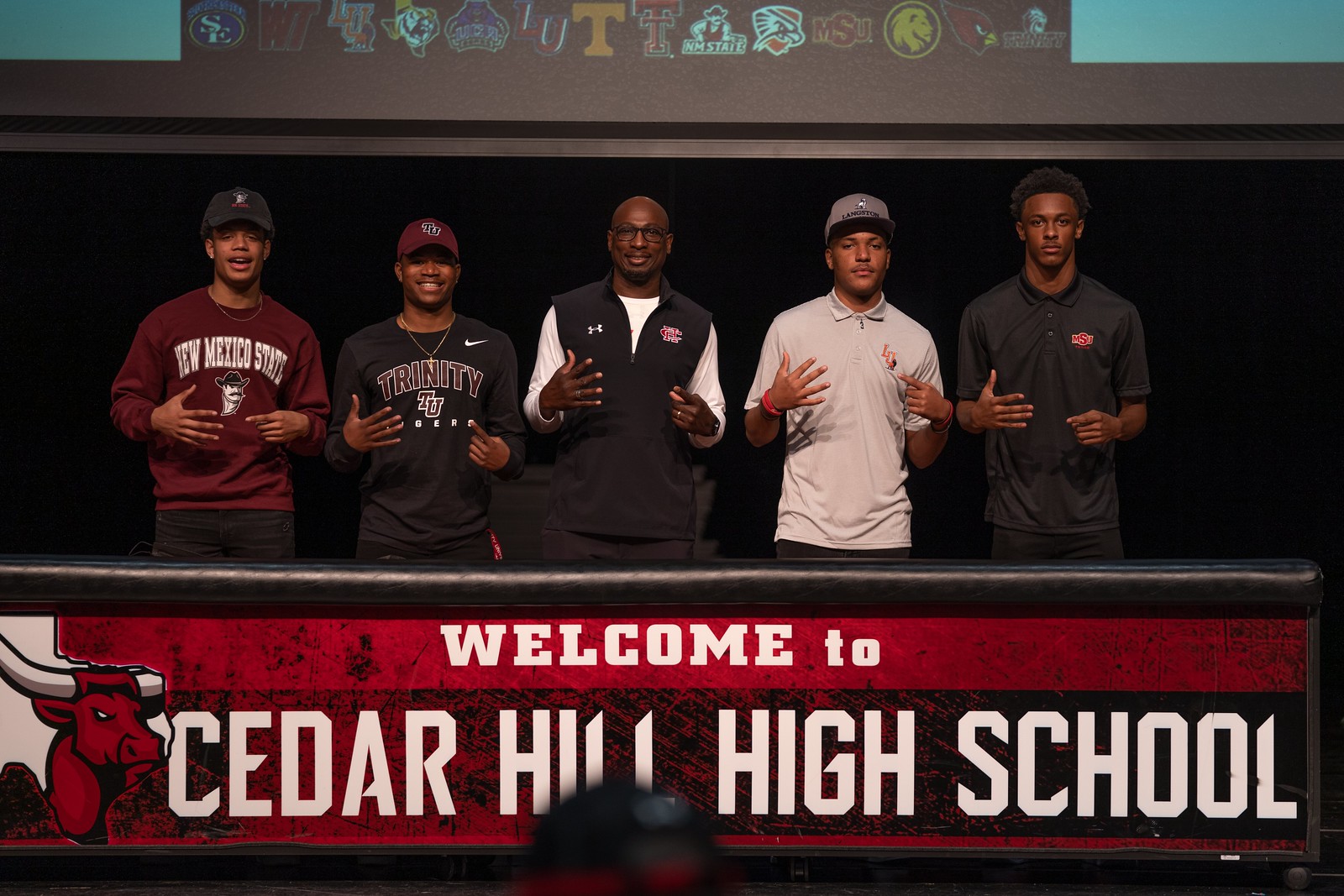In this color photograph, five young men are standing together indoors against a predominantly black background. They are positioned closely in the center of the image, with the three on the left smiling and the two on the right maintaining a neutral expression. Four of the men are wearing baseball caps, while one is not. They are dressed in a combination of black, white, and maroon clothing. Each has their hands held out in front of them, with their right hand pointing toward their left hand. 

Below them is a long table adorned with a maroon banner that reads "Welcome to Cedar Hill High School" in white text. To the left of the banner, a small mascot resembling a bull can be seen. At the top of the image, a screen is partially visible, adding to the indoor school setting. The background is a mix of black and red, tying the elements together with a contrast of colors that also includes hints of gray, blue, orange, and yellow.